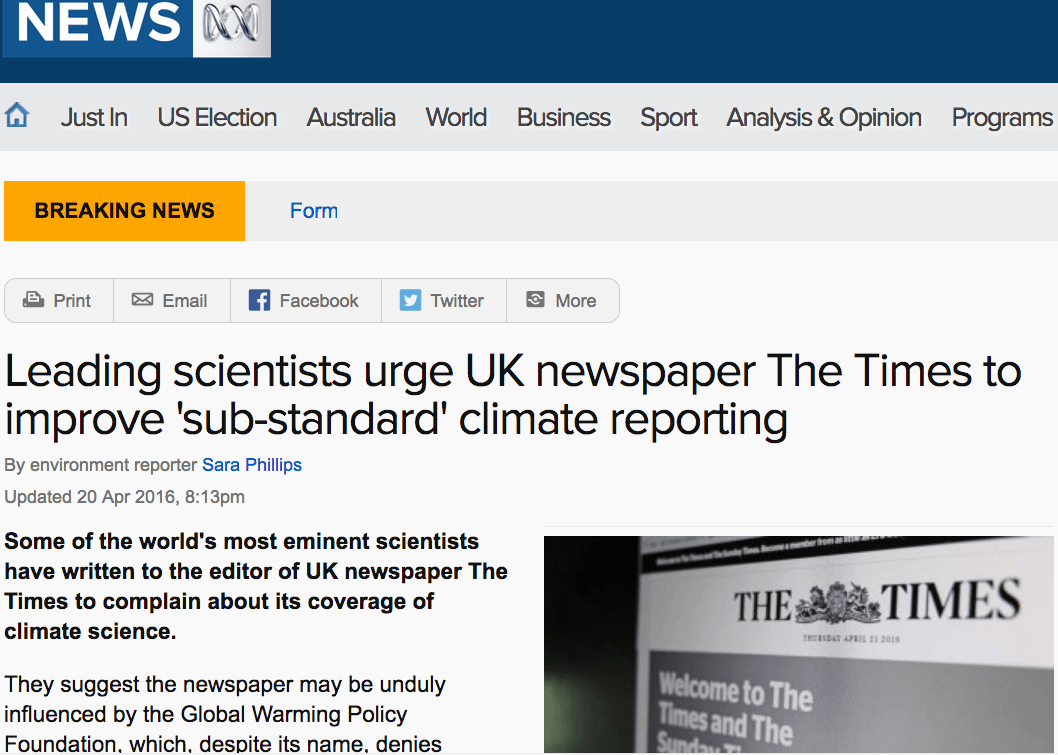This is a detailed screenshot of a news webpage. In the top right-hand corner, the word "News" is prominently displayed in white text. Directly below this is a "Home" button, and to its right, a horizontal navigation menu featuring categories such as "Just In," "U.S. Election," "Australia," "World," "Business," "Sport," "Analysis and Opinion," and "Programs." Below this navigation menu, set against an orangish-yellow background, the words "Breaking News" stand out.

The main headline reads, "Leading scientists urge U.K. newspaper, The Times, to improve substandard climate reporting." The article begins with the statement, "Some of the world's most eminent scientists have written to the editor of U.K. newspaper, The Times, to complain about its coverage of climate science. They suggest the newspaper may be unduly influenced by the Global Warming Policy Foundation, which, despite its name, denies..." The text cuts off here at the bottom of the picture.

In the lower right corner of the page is a photograph. This image appears to be either the front page of a newspaper or the door of an office. It prominently features "The Times" in large text, with a stylized logo between the two words that is difficult to read due to blurriness. Below "The Times," the date "Thursday, April 21, 2016" is visible, though slightly unclear. Beneath the date, incomplete text reads, "Welcome to The Times, and the Sunday," before it too cuts off.